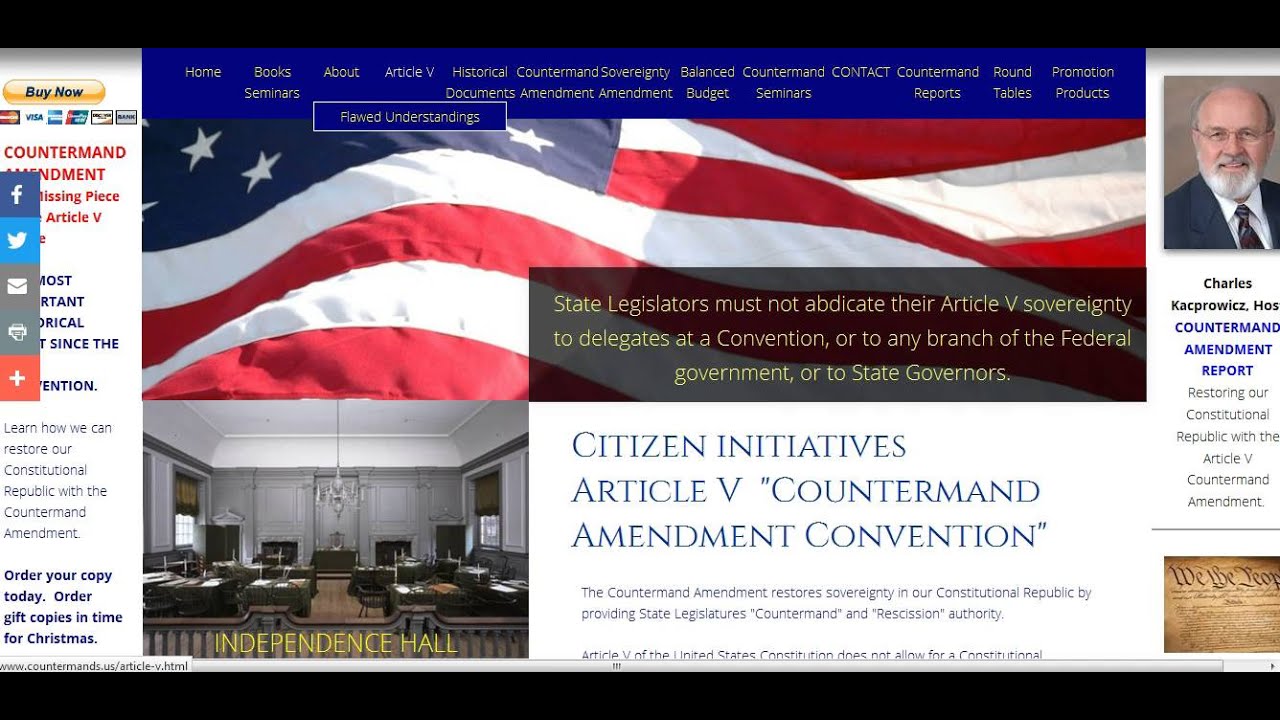The website exudes a patriotic theme, prominently featuring the national flag in a partially visible background image that complements the overall design. At the top of the page, the navigation menu includes links to various sections: "Home," "Books," "Seminars," "About," "Article 5," "Historical Counterman's Sovereignty," "Amendment Document," "Balanced Budget," "Counterman's Seminar," "Contact," "Counterman's Report," "Roundtable," and "Promotional Products."

Overlaying the image of the flag is a bold statement: "State legislators must not abide by Article 5 sovereignty to delegate at conventions or to any branch of the federal government or to any state." Below this, on a white background, is another phrase: "Citizens Initiatives Article 5 Counterman Amendments Convention."

On the left side of the website, there is a "Buy Now" section, featuring payment options such as MasterCard, Visa, American Express, Discover, and others that are not recommended. Adjacent to this, the text "Counterman Amendment," along with additional information about Article 5, is somewhat obscured by a social media toolbar. This toolbar includes icons for Facebook, Twitter, Email, Print, and Google+, partially covering the text on the left side of the page.